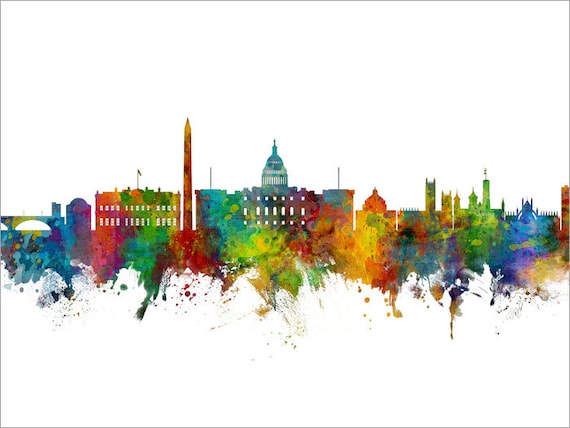This artwork is a vibrant, colorful watercolor painting capturing the essence of the Washington, D.C. skyline on a white canvas. Most of the canvas remains blank, accentuating the vivid scene concentrated in the center. The painting features major architectural landmarks such as the Capitol, the White House, and the Pentagon, as well as other significant buildings. Interestingly, the painting includes a mélange of iconic structures from around the world, like London's Big Ben, blending them into the D.C. landscape.

The color palette is diverse, encompassing a spectrum of rainbow hues from red, green, and blue to orange, yellow, and purple. These colors are splashed together in a dynamic and abstract fashion, creating a lively and chaotic lower portion of the buildings. The upper outlines of the buildings, however, are precisely defined, providing a stark contrast against the vibrant, messy splatters below, making this piece an intriguing blend of structure and spontaneity.